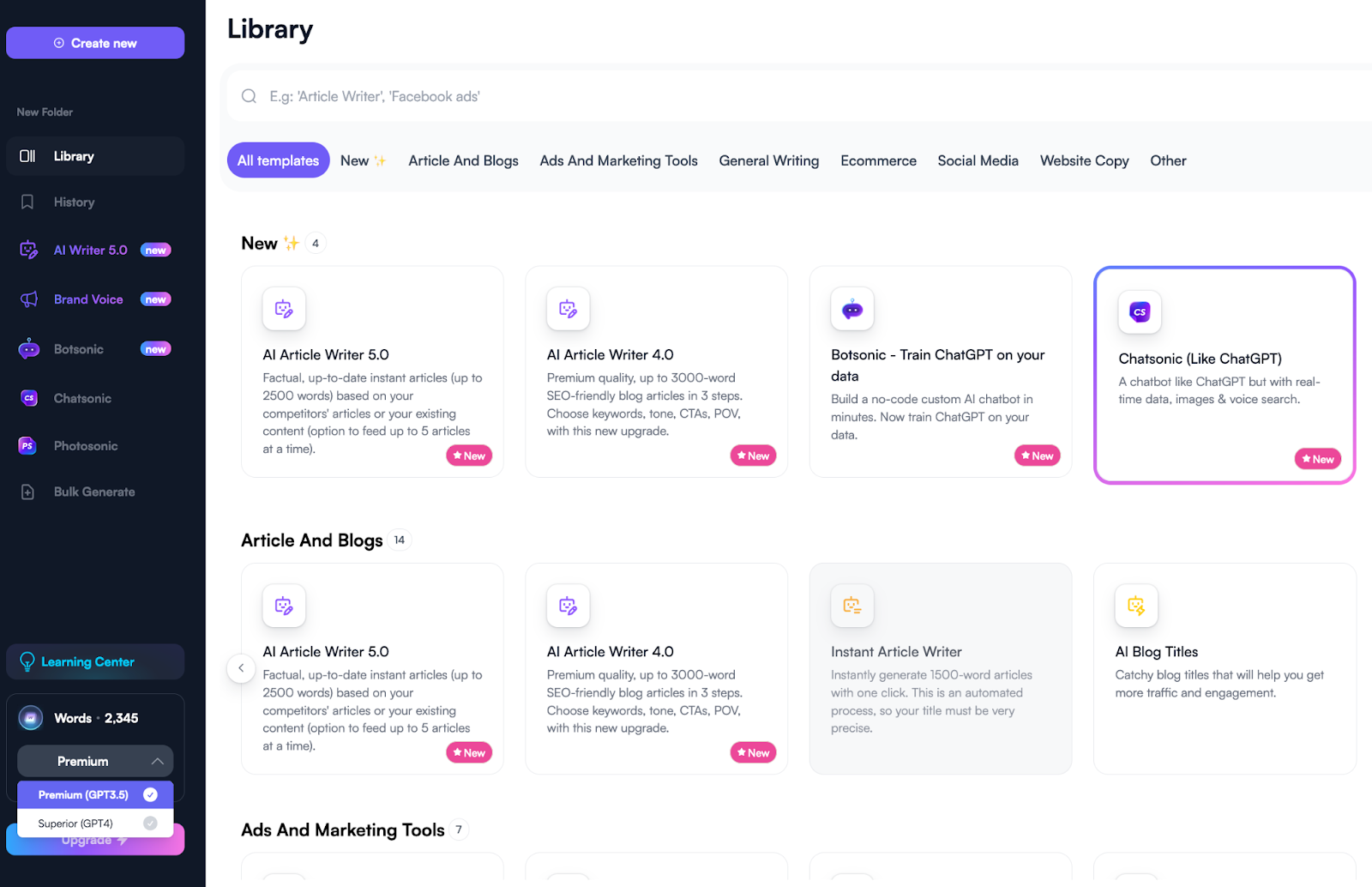The image features a user interface with a variety of elements. On the left side, there is a vertical black bar containing navigational options. At the top of this bar is a prominent blue button labeled "Create," followed by the word "Library." Lower on the bar, there are additional unreadable options, culminating in a "Learning Center" label at the bottom. Adjacent to the "Learning Center" is a black button marked "Premium." Further down are two buttons—one blue and one white—each containing unreadable text.

On the right side of the image, set against a white background, is the header "Library." Directly below this header is a search bar. Beneath the search bar are eight distinct squares, each featuring an icon on the left and associated text. The readable segments of these texts include labels such as "AI Article Writer 5.0," "AI Article Writer 4.0," "Train Chat GPT on Your [unreadable]," "Chat Sonic Live Chat GPT," and "AI Blog Titles."

The layout suggests a dashboard or interface related to AI-driven content creation tools and educational resources.